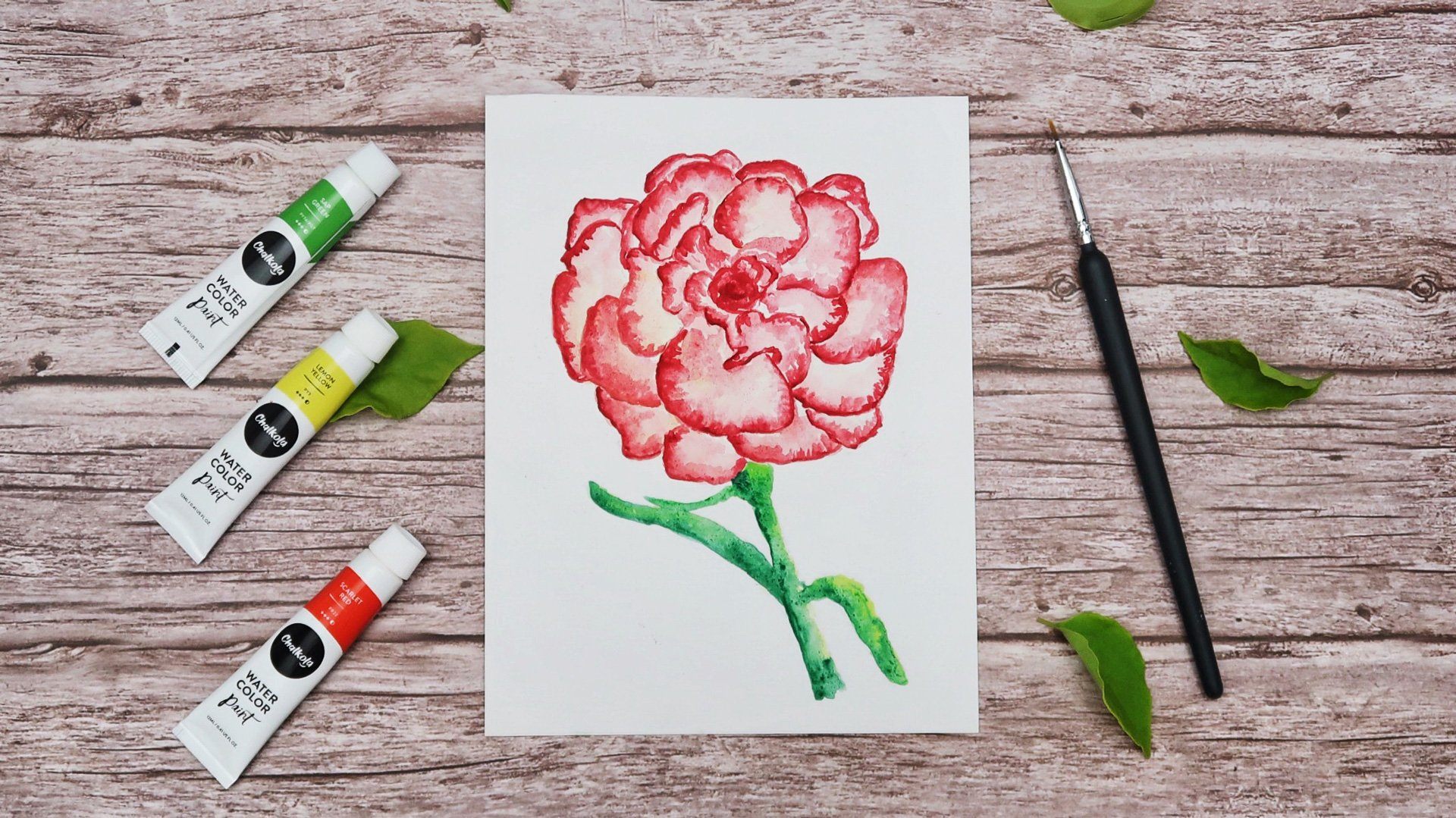This image depicts a carefully arranged scene on a light grayish wooden table, showing off grains of the wood. At the center of the table lies a vertically-placed white piece of paper featuring a simple yet detailed watercolor painting. The painting portrays a flower, possibly a rose, with green stems and a mix of pinkish-red and reddish petals, accented with touches of white to lighten the red in places. The painting also includes green leaves on either side of the stem.

To the left of the paper, there are three neatly aligned white tubes of watercolor paint, each marked with a stripe indicating its color content—green, yellow, and red respectively. Each tube features a small black circle and a green leaf motif under the yellow portion, emphasizing the natural colors used in the painting.

On the right side of the paper lies a slender paintbrush, approximately the same length as the sheet. The brush features a black handle and a silver tip with bristles protruding from the end, ready for future artistic endeavors. The composition, viewed from above, showcases the artist's tools and their creation in a harmonious, aesthetically pleasing arrangement.